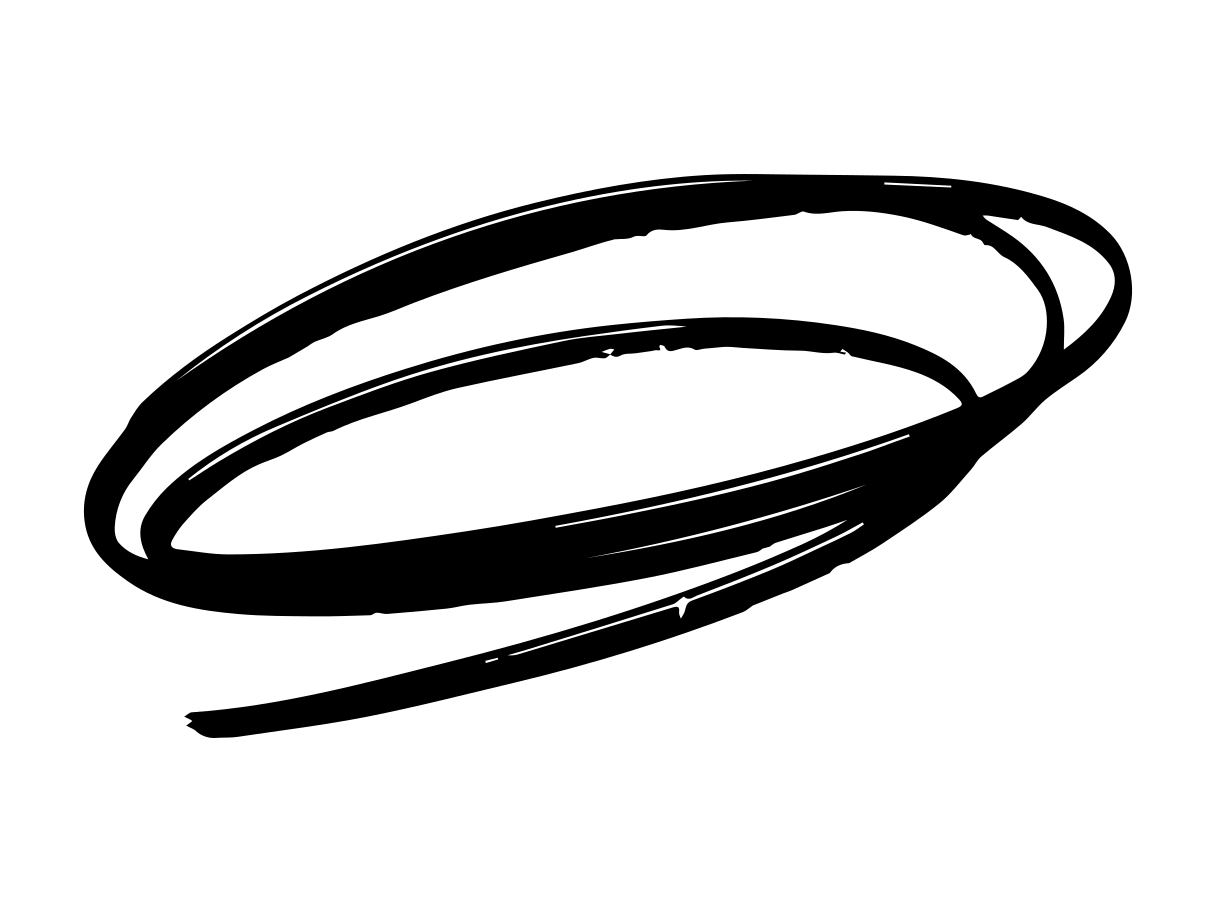The image features a simplistic yet dynamic black spiral doodle against a solid white background, reminiscent of a loosely coiled wire or a spring. The irregular, overlapping ovals create an impression of energetic, spontaneous movement, as if someone had whimsically drawn multiple circular shapes freehand with an ink pen or marker. The design, devoid of any connectors or text, exudes a raw, unrefined charm with scattered white specks adding to its organic feel. This black squiggle, shiny and thicker than typical twine, coils upon itself about four or five times, conjuring up images of a tornado viewed in mid-formation. The overall effect is one of improvisation and liveliness, captured with an intentional simplicity that evokes both the potential of a logo and the carefree nature of a random doodle.